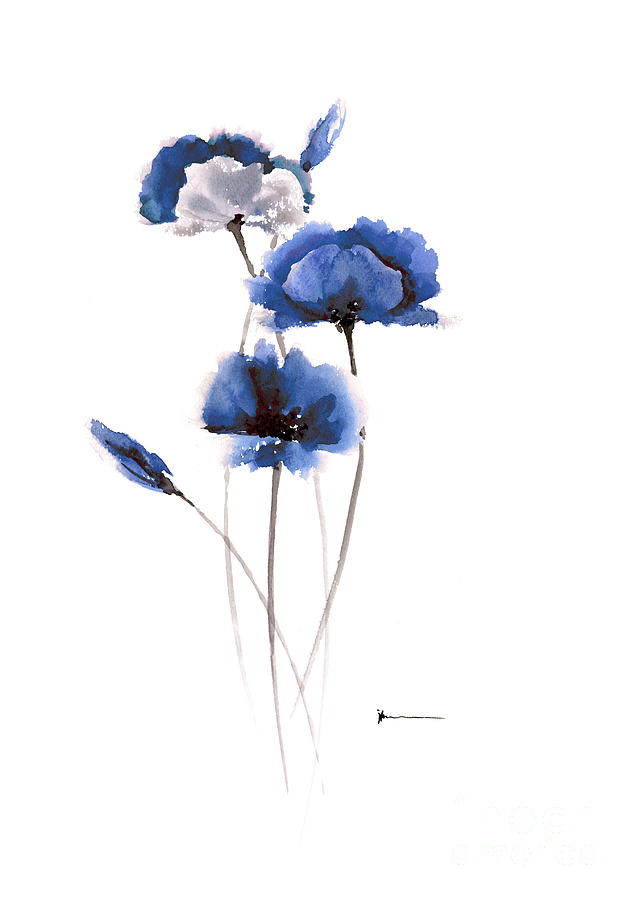This image presents a detailed watercolor painting set against a plain white background. The artwork features a collection of blue and white fan-shaped flowers with subtle black accents and thin, gray painted stems. The floral arrangement includes fully bloomed flowers as well as a couple of buds yet to open, adding to the composition's dynamic nature. One of the flowers distinctly incorporates both blue and white hues, providing a fleck of contrast within the predominantly blue palette. The flowers exhibit a round, fluffy appearance, characteristic of the watercolor technique where colors spread softly. On the bottom right of the image, there's a dark, slightly squiggled black line, which might mistakenly suggest a signature but actually appears as just an abstract stroke. The overall painting showcases a delicate interplay of colors and textures, capturing the ethereal essence of watercolor art.